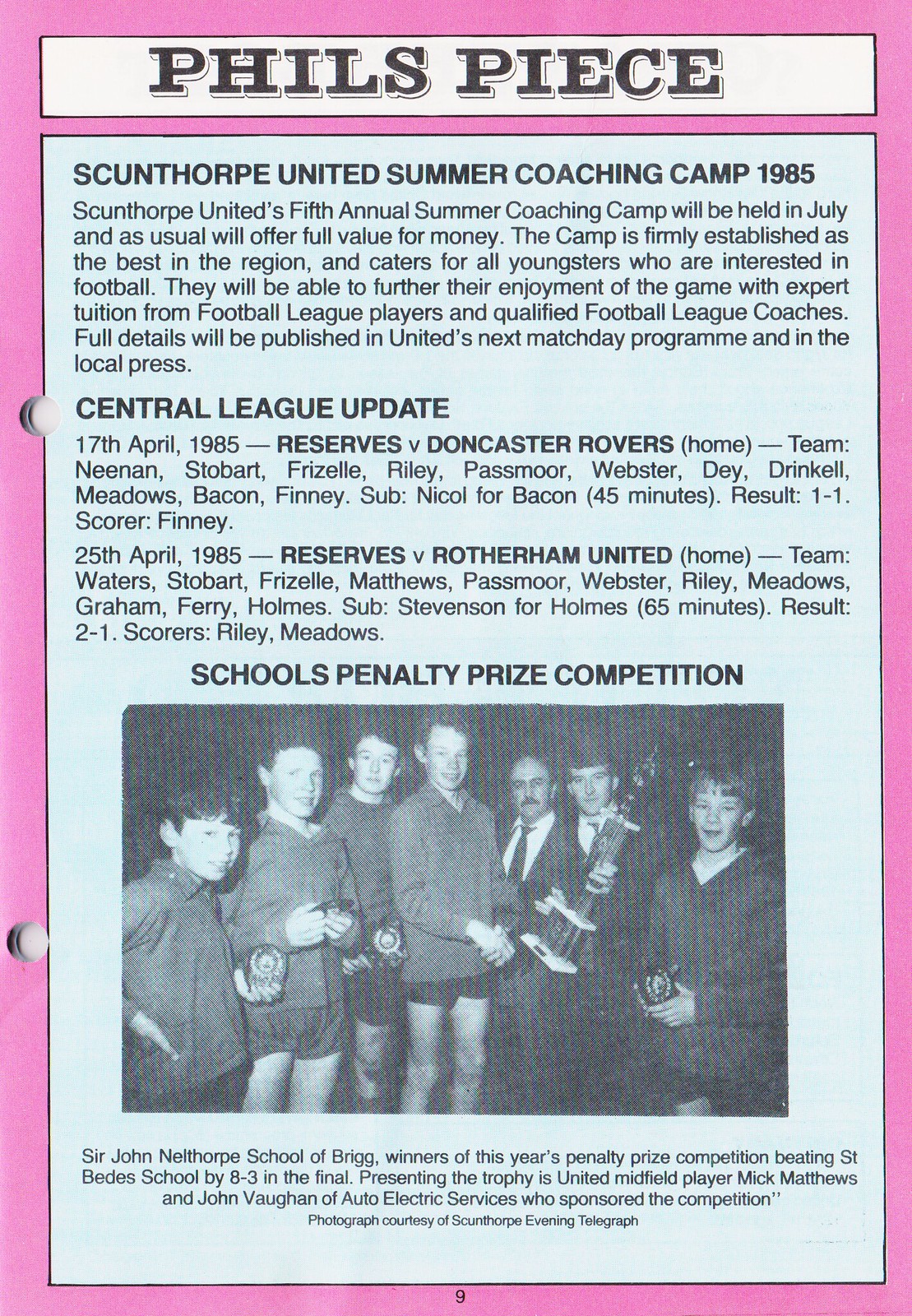The image depicts a monochrome photograph set against a purple pamphlet background with a gray label containing various texts. The main title reads "Feels Peace" and the pamphlet is for the "Scunthorpe United Summer Coaching Camp 1985". The photograph shows a group of schoolboys and two adults. There are five schoolboys in total: three on the left, then the two adults, and one boy on the right. Four boys are clearly wearing shorts and jackets, and one boy's attire is partially obscured but also seems to include a jacket. The adults are dressed in sports suits and ties.

In the photograph, one of the adults, identified as United midfield player Mick Matthews, is holding a trophy, alongside John Vaughan of Auto Electric Services, who sponsored the competition. The text below the photograph describes this as the "Sir John Netthorpe School of Brig, winners of this year's penalty prize for competition, beating St. Pete's School by 8-3 in the final."

The pamphlet also includes text about the upcoming Scunthorpe United's fifth annual summer coaching camp to be held in July 1985, emphasizing the camp’s reputation as the best in the region, offering expert tuition and full value for money. Additionally, there are Central League updates detailing match results from April 1985, including match scores and team listings.

This detailed caption covers the dual aspects of the pamphlet: promoting the summer coaching camp and celebrating the schoolboys' sporting achievements.